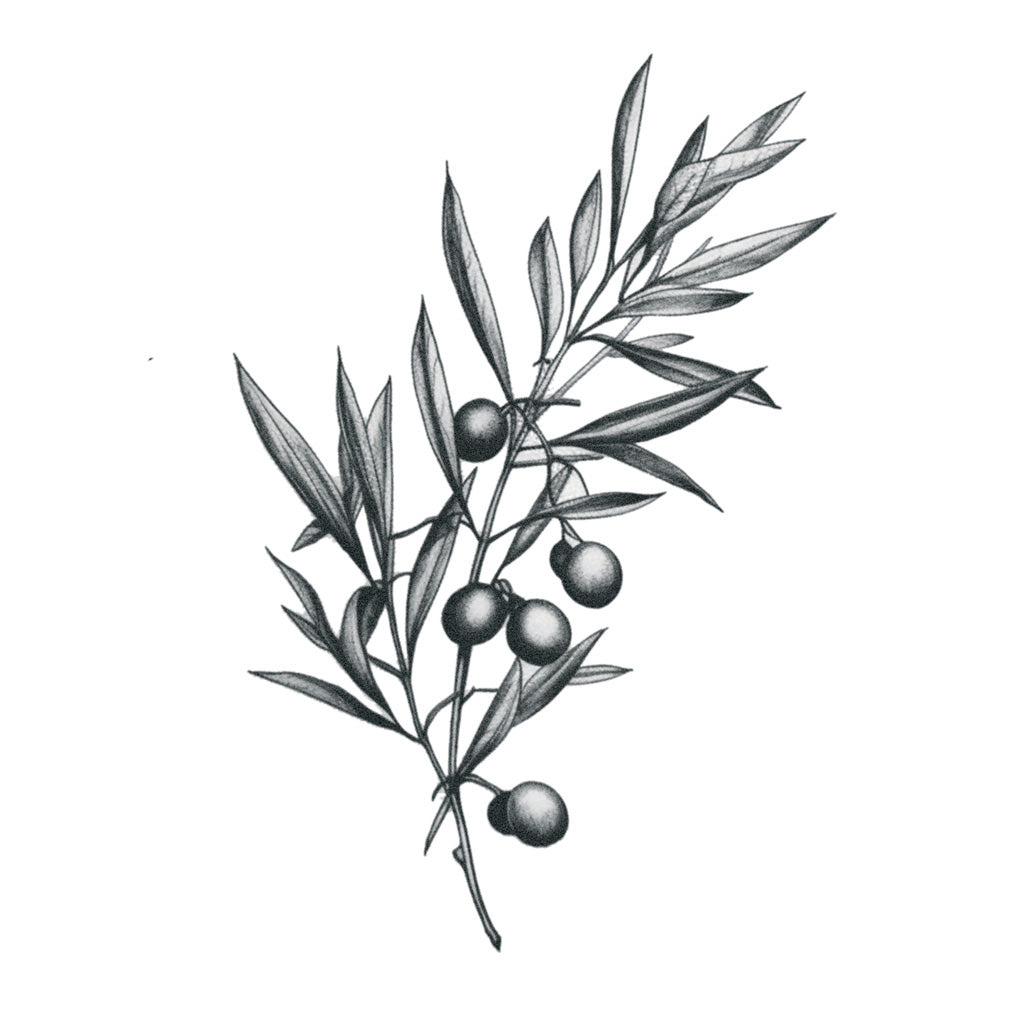The image is a detailed black ink drawing set against a plain white background, depicting an herb-like plant. Central to the illustration are two interconnected plant stems adorned with long, thin, and pointed leaves that sometimes fold over. Branching from the stems are small round fruits that resemble either olives or cherries, with distinct smaller circles on top of them. There are six of these fruits in total, some partially hidden behind others. The illustration focuses on the stems, leaves, and fruits in clear black ink, without any other distracting elements or background.